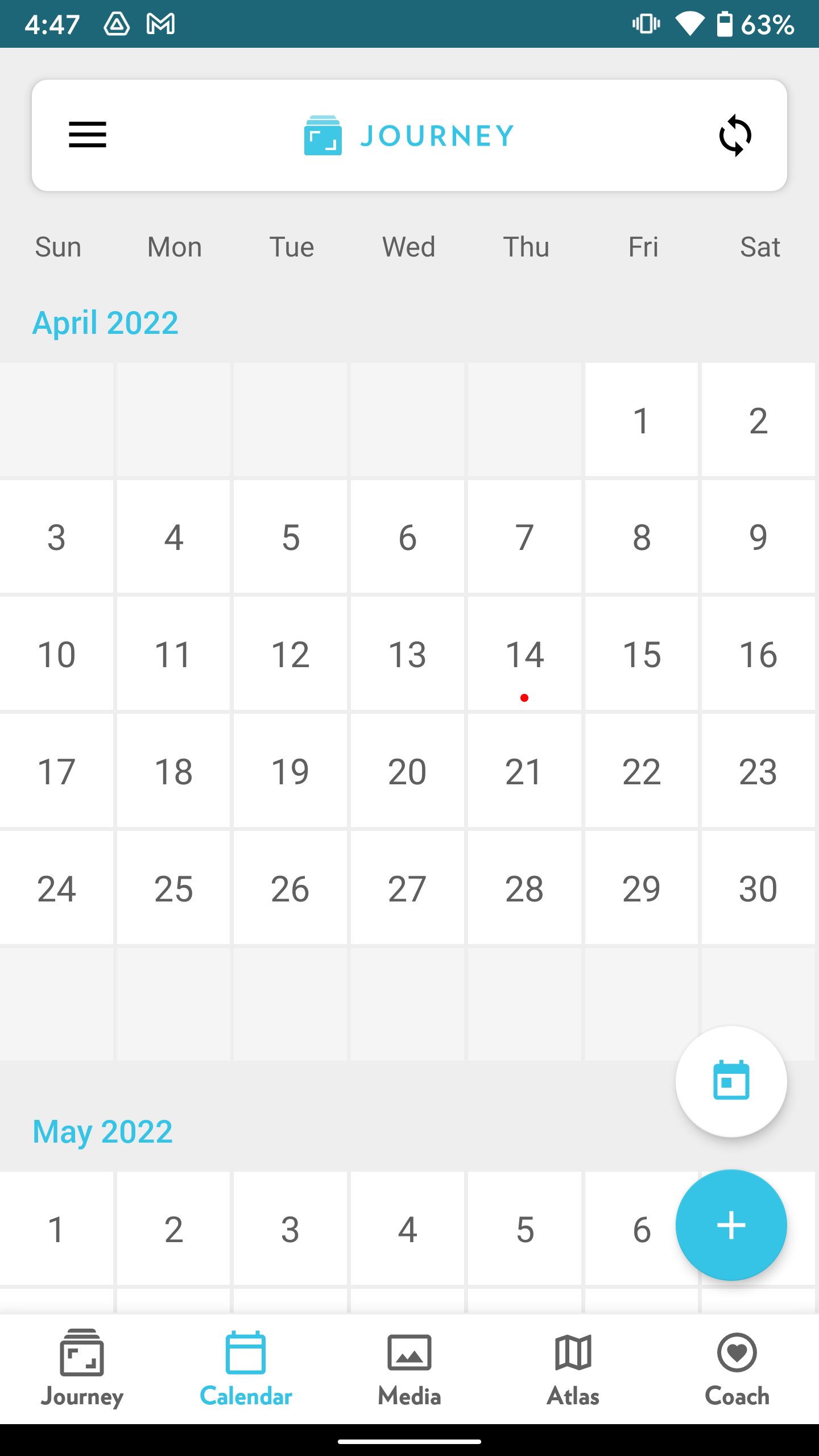The image is a screenshot from a smartphone displaying a calendar app named "Jane." At the top of the app, the name "Jane" is prominently written in blue with two icons flanking it: a settings icon on the left, represented by three horizontal black lines, and a refresh icon on the right, depicted as two circulating black arrows. 

The open month on the calendar is April 2022, with a sneak peek of May 2022 visible at the bottom. Both month names are written in blue, while the days of the week, spanning from Sunday to Saturday, are marked in gray. Notably, there is a red dot beneath the 14th of April, indicating an event on that day.

In the bottom left corner of the app, there is a blue circular button with a white plus sign, and directly above it, there is another button designed as a calendar icon colored in white and blue. The app interface includes a navigation bar at the bottom featuring five tabs: "Jane," "Calendar," "Media," "Atlas," and "Coach." Except for the "Calendar" tab, which is highlighted in blue, the other tabs are displayed in gray.